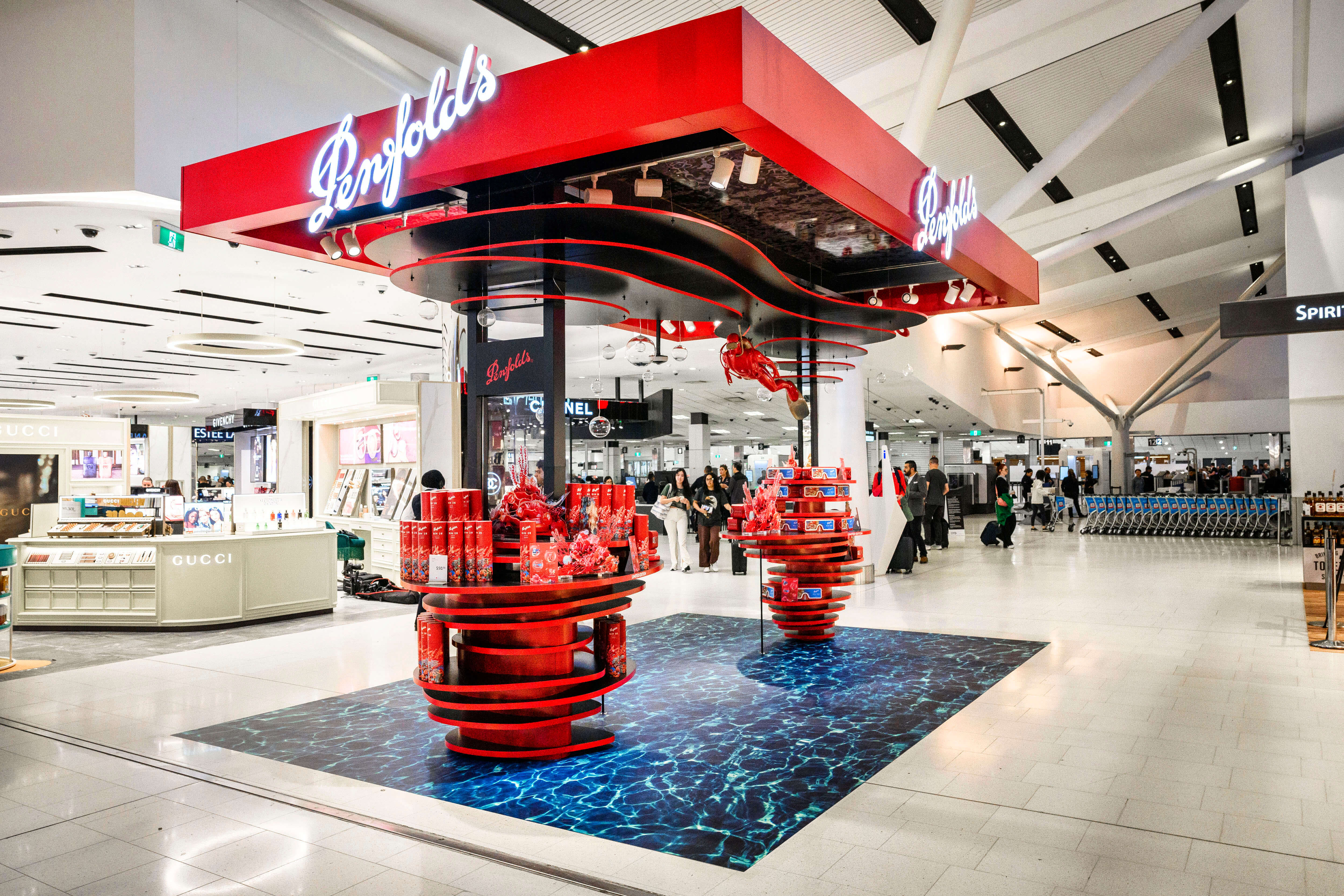The image appears to be taken inside a large, bustling space that could be either a shopping mall or an airport. In the foreground, there is a striking kiosk. The kiosk has a prominent red roof supported by two black pillars, with "Penfolds" written in stylish cursive, white font on all visible sides. Under the roof, two circular red counters display various red cylindrical and square products. The floor directly beneath the kiosk has a unique blue and black pattern, resembling water, with a figure-eight shape outlined in red.

Surrounding the kiosk, the floor transitions into a light-colored tile. To the left, there is a pristine white store with the word "Gucci" prominently displayed on the front of its octagonal counter. Further to the right, a sign reading "Spirit" in white font against a black background suggests the presence of Spirit Airlines, hinting that this might indeed be an airport. In the background, many people are milling about, some appearing to wear uniforms with black tops and white pants, adding to the busy atmosphere. There is also a line of shopping or baggage carts to the right, characterized by blue shelves and an aluminum frame. Overall, the setting is lively with a blend of retail and possible travel elements.